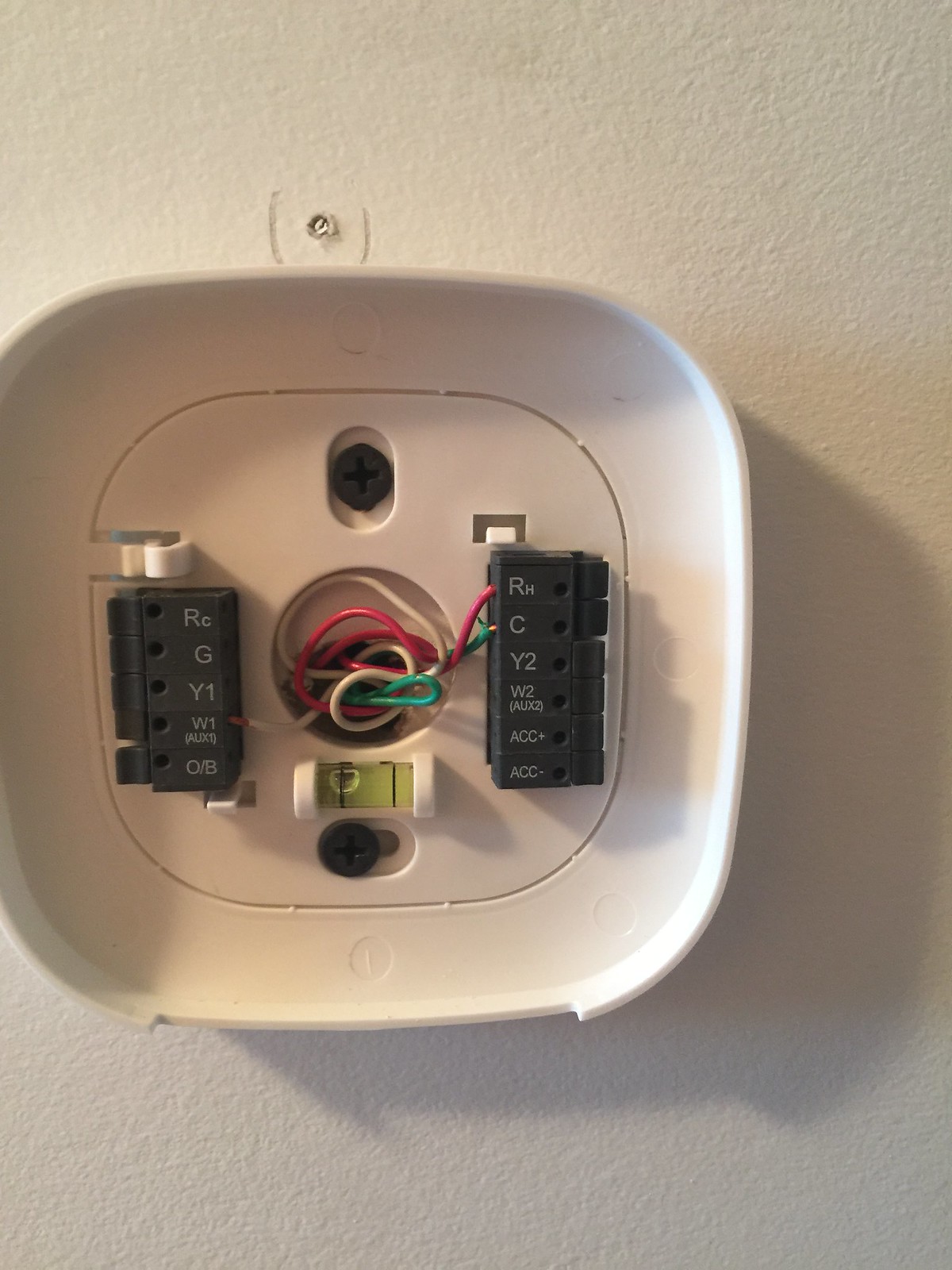The image depicts a disassembled electronic device, somewhat resembling a smoke alarm, mounted on a wall. The faceplate has been removed, revealing the intricate internal components. Multiple colored wires are visible, connecting to two distinct computer chips. The chip on the left has the labels "RCGY1W1" and "auxiliary O/B," while the chip on the right is marked "RHCY2W2" and "ACC + ACC -," which appear to signify different electronic functions or supplies. Intriguingly, there is a small liquid-filled level with a bubble, commonly used to ensure proper alignment, nestled beneath the wires. Despite its complex appearance, the exact purpose of this device remains unclear.